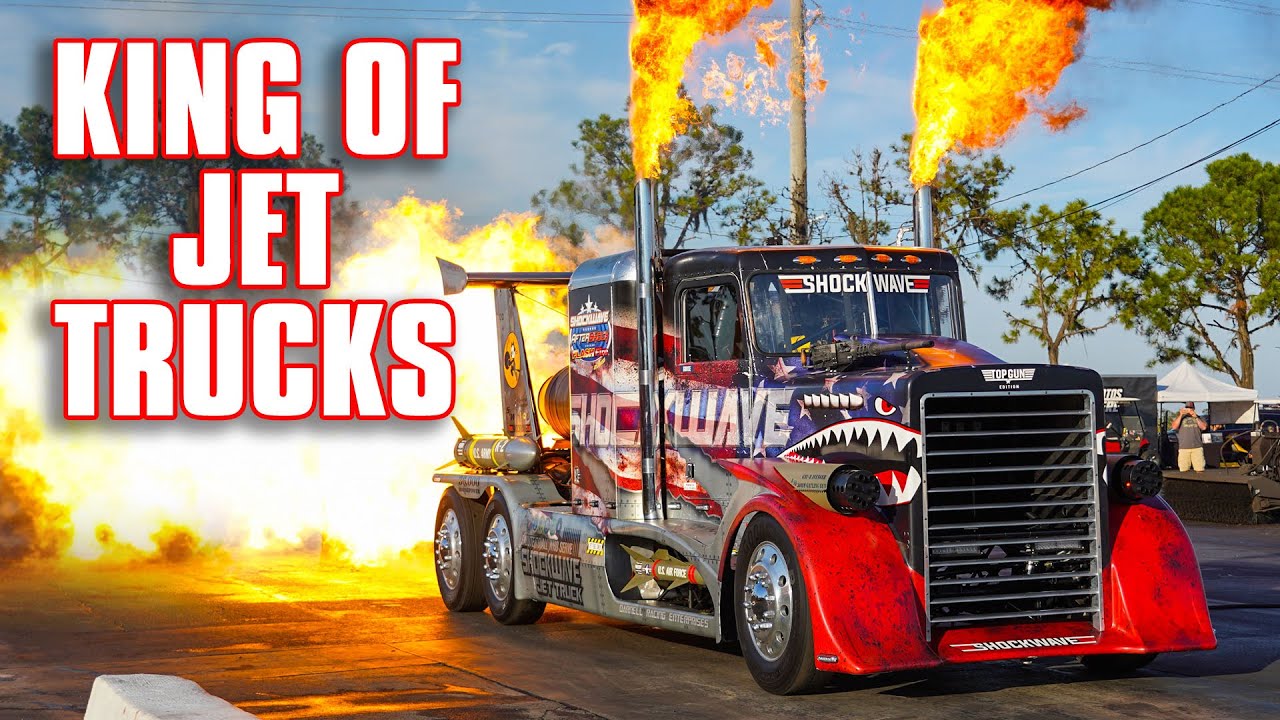Behold the "King of Jet Trucks": Shockwave, a monstrous, jet-powered truck that looks as if it could rocket into the stratosphere. Dominating the image is a colossal truck, painted with striking red and dark blue hues, adorned with intricate decals including a menacing shark eye and teeth near the grill. The truck boasts a pair of massive, silver exhaust pipes on each side just behind the cab doors, from which vibrant yellow and orange flames spectacularly burst forth.

Across the windshield in bold white letters is the name "Shockwave,” emphasizing its fearsome branding. At the back, a menacing rocket is mounted above the rear fender, adding to the truck’s larger-than-life persona. A giant spoiler and tall stabilization fins at the rear frame the fiery inferno that trails behind, suggesting sheer, unrestrained power. The text "King of Jet Trucks" is emblazoned to one side in striking white letters, outlined in red, reinforcing its title.

With fire shooting into the sky and a background ablaze with flames, this awe-inspiring machine appears to be powered by a jet engine, symbolizing raw, unstoppable force.